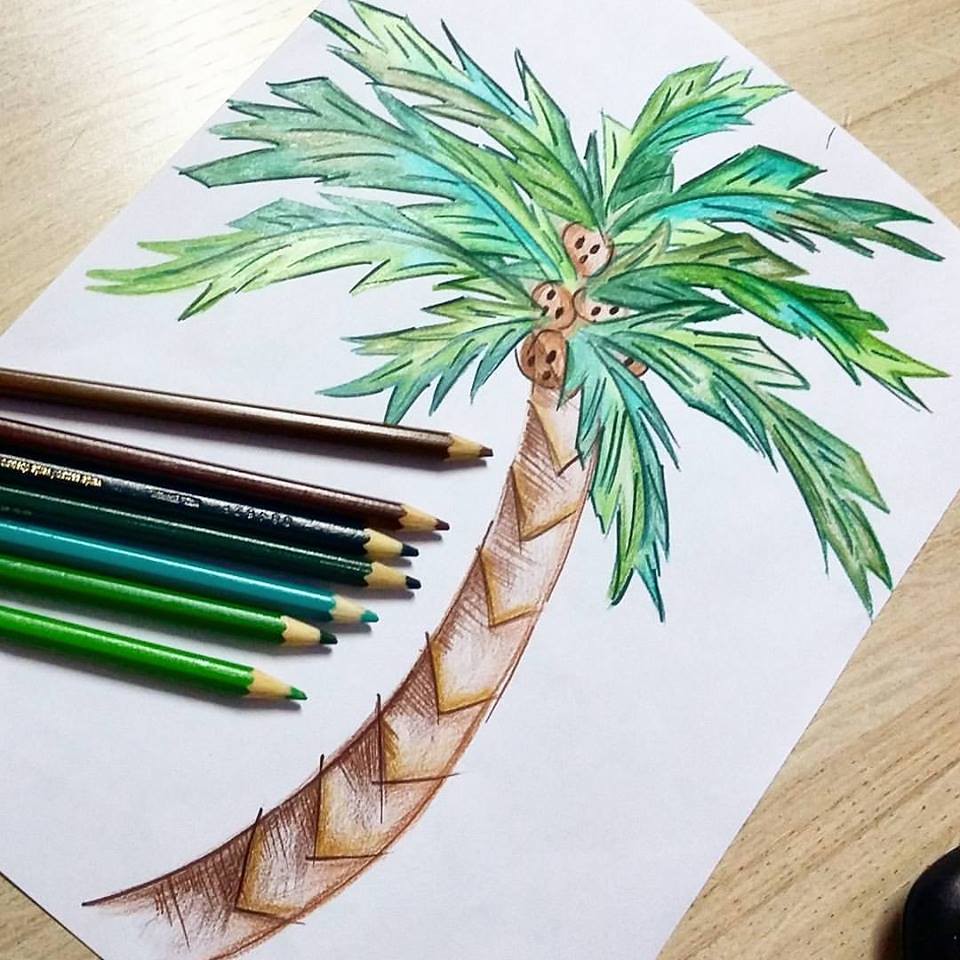This detailed photograph showcases a colored pencil drawing of a palm tree on a white piece of printer paper, which is placed diagonally on a light brown wooden table. The palm tree, drawn in a high-quality yet not entirely realistic style, features a slightly curving brown trunk and numerous detailed palm fronds in various shades of green. Nestled among the leaves are several coconuts, also shaded in brown. Seven colored pencils, presumably used in the creation of the drawing, are meticulously arranged to the left of the paper. From bottom to top, the pencils include a light green, medium green, blue-green, dark green, dark blue, light brown, and dark brown. The entire setup is captured in a well-composed image, angled such that the tree base starts in the bottom left corner and extends upward.